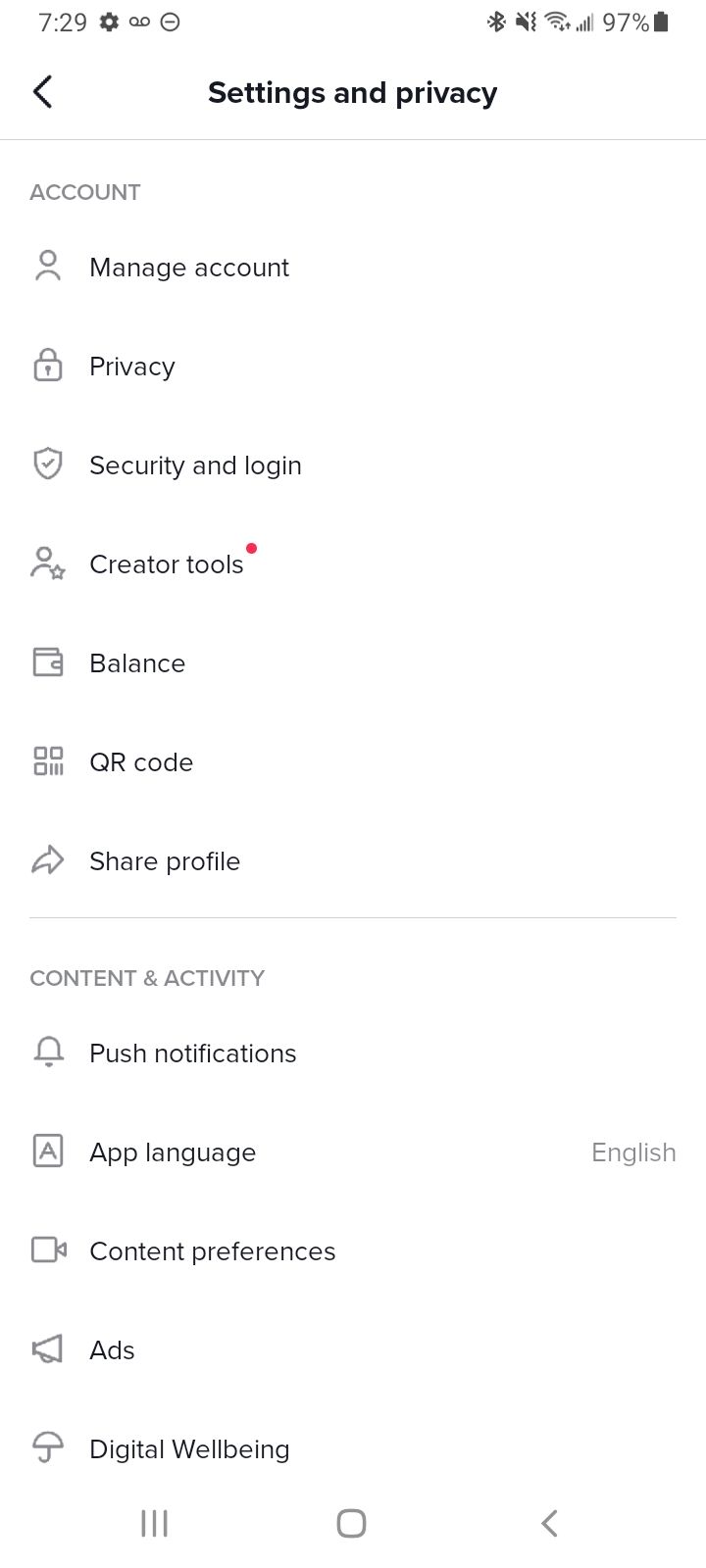A smartphone screen displays the "Settings and Privacy" section of an application. At the top, the status bar shows the time as 7:29, along with icons indicating that the microphone is off, the Wi-Fi connection is active, and the battery is nearly full. Below this, a back arrow at the top left suggests an easy return to the main settings menu.

The screen is divided into two main sections. The first section is labeled "Account" and includes options such as "Manage Your Account," "Privacy," "Security and Login," "Creator Tools," "Balance," "QR Code," and "Share Profile." Notably, "Creator Tools" has a small red dot beside it, potentially indicating new features or unread notifications within.

A separator line divides the account section from the "Content and Activity" section. Here, users can access "Push Notifications," "App Language," "Content Preferences," "Ads," and "Digital Wellbeing." Among these, only "App Language" has a selectable option displayed, which is currently set to English.

At the bottom of the screen, typical navigation buttons are shown: three vertical bars that are likely for the app's main menu, a square that typically represents the home button, and a left-facing arrow on the right, which allows users to go back to the previous page.